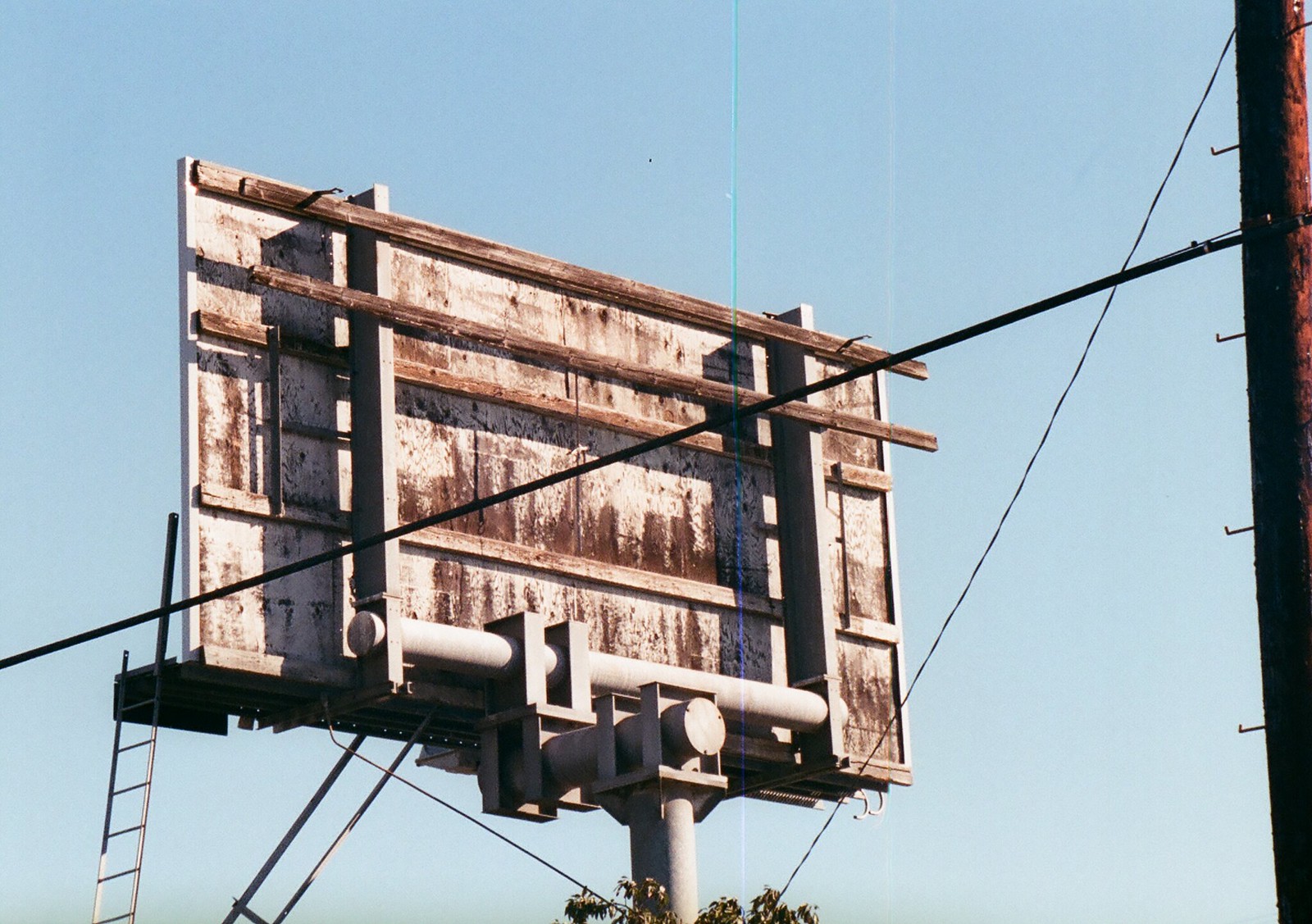This outdoor digital photograph captures the back side of a weathered billboard, supported by a large metal pipe rising from the ground. The billboard, primarily light gray with sections obscured by extreme rust, features several exposed beams and metal struts extending vertically from a rounded crossbar. Some of these beams are distinctly wooden, adding to the aged and decayed appearance. A metal ladder hangs off the left edge of the billboard, leading up to its platform. 

In the foreground, various cables and support wires, including some likely originating from a brown wooden telephone pole on the right side of the image, stretch at angles across the scene. The telephone pole is fitted with black metal climbing hooks evenly spaced along the left side. About three-fourths up this pole, a significant black cable runs diagonally toward the bottom left, accompanied by a smaller cable extending from the top down to near the bottom center of the frame.

In addition to these elements, the tops of green-leaved trees peek out at the bottom of the image, contributing a touch of nature to the industrial scenery. Above, the sky is a bright blue without any visible clouds, suggesting a clear day. The overall structure of the billboard appears over-engineered, hinting at its old yet robust design.